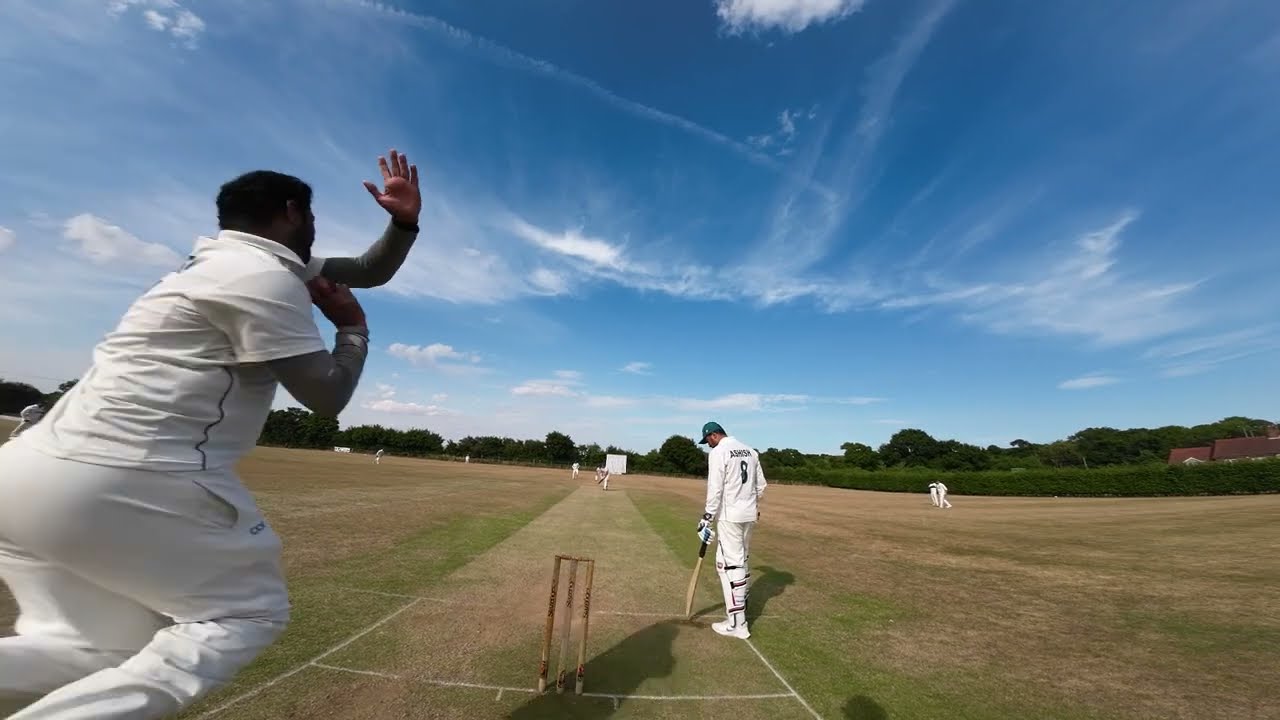The image depicts a tense moment in a cricket match being played on a vast, green field bordered by a tree line under a blue sky scattered with feathery white clouds. Central to the scene are two players in action: to the left, a man mid-throw with one hand extended back, preparing to deliver the ball, and to the right, another man poised with a cricket bat held in his left hand. Both players wear white jumpsuits adorned with black numbers and letters, notably '8' on the back of one player's shirt. Near the wickets and the cricket paddle, which is brown with a black handle, the grassy ground varies in hues of green and brown. In the background, other players in similar white attire can be vaguely seen, further emphasizing the active sporting event. The serene landscape is completed with the presence of a building featuring a red roof and white sidings peeking in from the right, harmonizing with the natural and sporting elements of the picturesque cricket match.